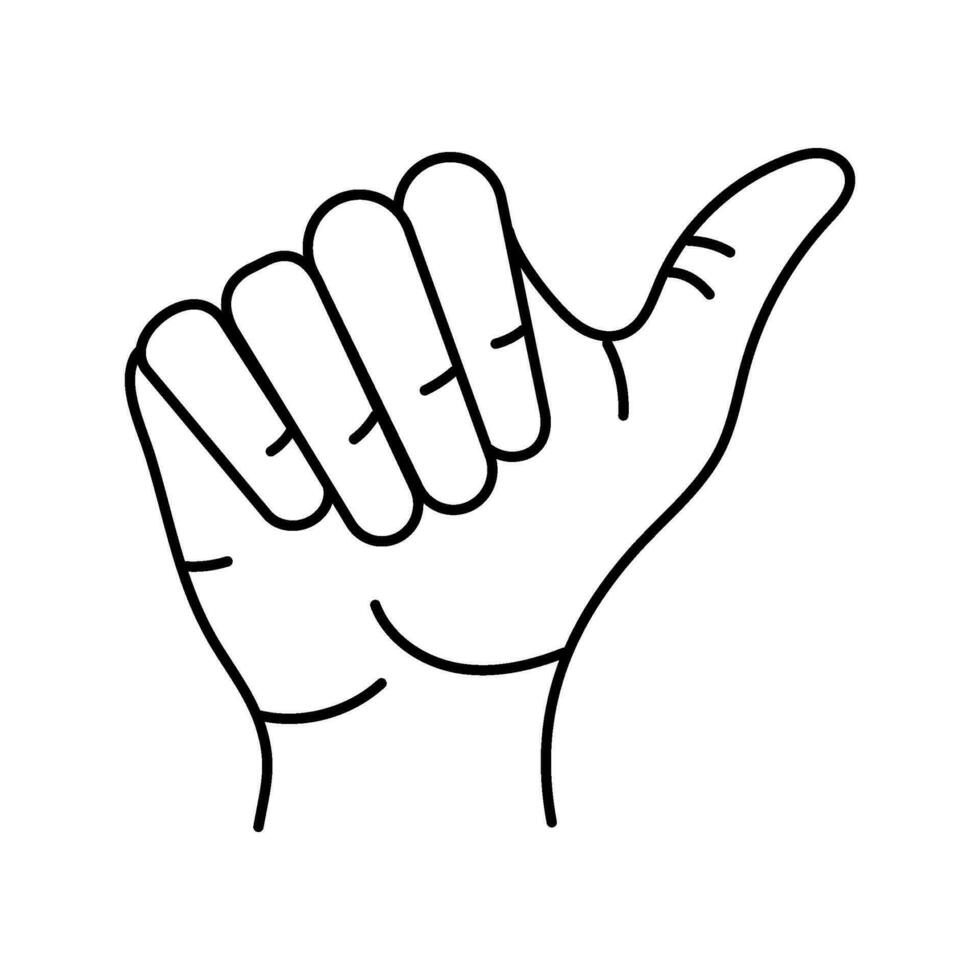A simplified, black line drawing depicts a right hand on a white background, creating a striking contrast. The hand is cupped with elongated fingers clenched over the palm, and the thumb extended outward as if in a hitchhiking gesture, pointing towards the two o'clock position. Despite its minimalistic style, reminiscent of a coloring book page or a digital emoji, the image includes notable details like creases on each finger, the thumb, and the wrist. The prominent lines illustrate the separation between the thumb and forefinger and emphasize the natural indentations and wrinkles of a human hand, giving it a slightly textured, three-dimensional appearance.